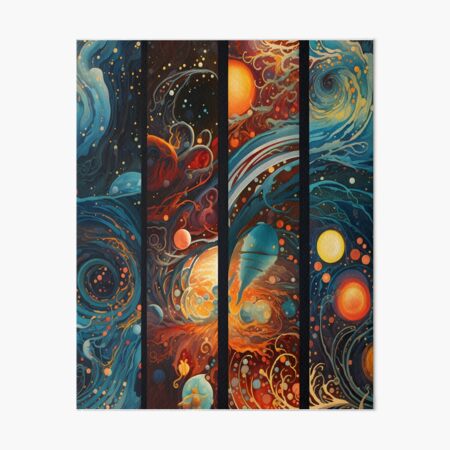The artwork is an intriguing composition of four vertically arranged rectangular panels, each contributing to a cohesive and vibrant display. The panels, either part of a single canvas split into sections or four canvases put together, share a common intergalactic and energetic theme, characterized by swirling patterns and a dynamic interplay of colors.

The leftmost panel features a dark blue color scheme with zigzag designs reminiscent of water waves, interspersed with a circular, snail-like shape adorned with red dots. This panel transitions into a second panel where mysterious black and red shapes dominate, highlighted by a vivid yellow circle and green vine-like elements.

The third panel introduces a predominantly orange background with a prominent half-circle at the top and a blue, carrot-like shape dangling near the bottom. This orange theme connects visually to the previous and following panels while maintaining its distinct color variations.

The final panel returns to a blue color scheme and features wave-like designs at the top. Below these, a light yellow and orange circle stands out, surrounded by medium and large spheres in yellow and orange.

Each panel is separated by a distinct black line, emphasizing the transition and flow from one to the next, yet maintaining an interconnectedness through the swirling and dreamlike patterns that extend across the entire composition. The overall effect is a mesmerizing blend of colors—reds, blues, oranges, yellows—creating a unified yet diverse visual experience that teems with motion and energy.